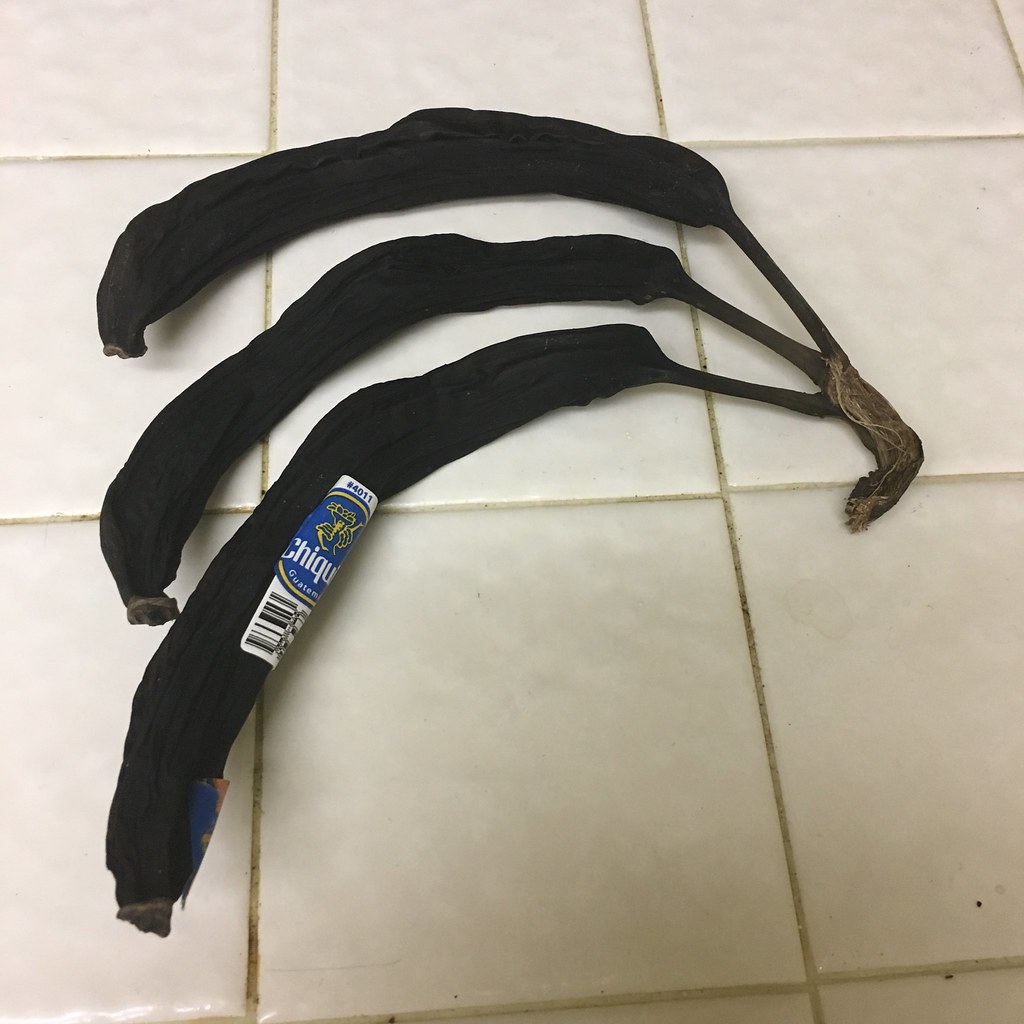This image captures a dismal indoor scene featuring three severely shriveled and blackened bananas laying on a noticeably unclean tile floor. Positioned side by side and still attached to their stem, the bananas lie with their bottoms to the left and stems to the right, stacked one on top of the other. The once-yellow fruits have dried to the point of resembling blackened string beans, devoid of moisture and visually unappealing. The bottom banana in the cluster sports a distinct Chiquita sticker with a barcode numbered 84011, still visible despite the decay. The floor beneath them is composed of off-white square tiles with dark grout that appears dirty and in need of cleaning. The tile layout is also remarkably uneven and poorly executed, adding to the overall state of neglect in the setting.